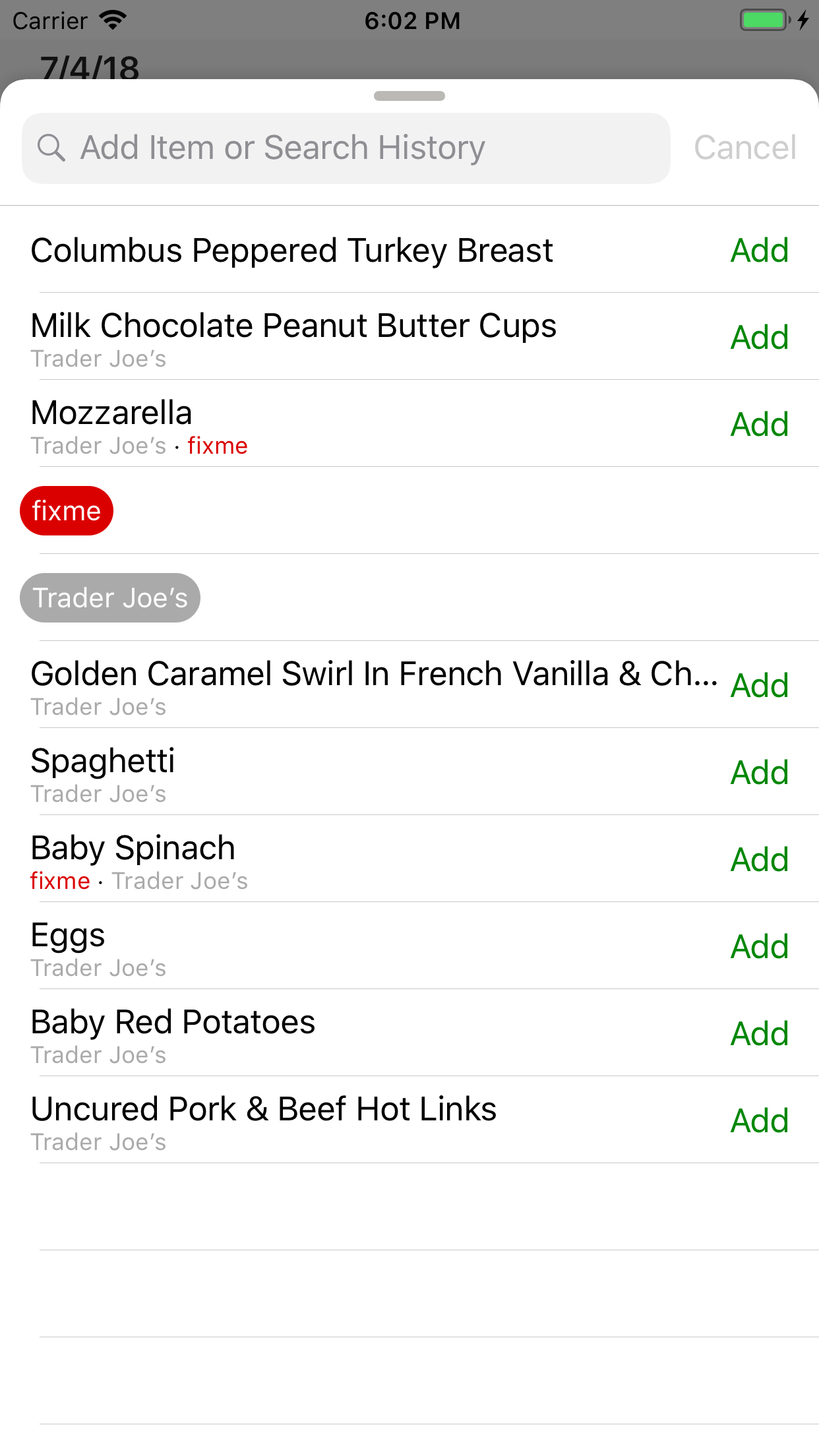A detailed description of the screenshot of the grocery list on a smartphone:

The image is a screenshot of a smartphone displaying a grocery list. At the top of the screen, the status bar shows the carrier name, a Wi-Fi symbol, the time "6:02 PM" centered, and a green battery icon with a small black lightning bolt, indicating that the phone is charging. The date displayed is "7/4/18."

Below the status bar is a search bar. Inside the search bar, the text "Add item or search history" is visible next to a small magnifying glass icon on the left. On the right side of the search bar, there is a "Cancel" button.

The grocery list itself starts below the search bar, with each food item listed in sequence. Each item on the list has an "Add" button in green to its right. The list begins with the following items:

1. Columbus peppered turkey breast
2. Milk chocolate peanut butter cups
3. Mozzarella (with "Trader Joe's" noted underneath this item)

There is a red oblong shape that says "fix me" below "Mozzarella," followed by a larger gray oblong shape that says "Trader Joe's." The list continues with:

4. Golden caramel swirl
5. French vanilla
6. Spaghetti
7. Baby spinach
8. Eggs
9. Baby red potatoes
10. Uncured pork and beef hot links

The screenshot captures a structured and detailed view of someone's grocery shopping list, emphasizing the organization and categorization of items, with some specified to be bought from Trader Joe's.